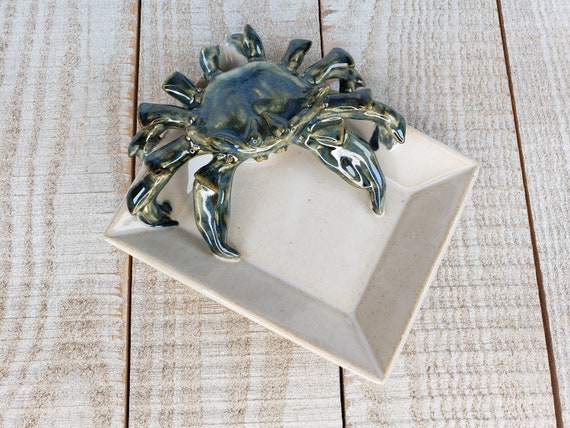This photographic image depicts a rectangular ceramic dish with an off-white glaze, positioned at a 30-degree diagonal from the bottom right to the top left. The dish, which could serve as an ashtray or a candy dish, features a striking metallic crab affixed to its top right corner. This crab, rendered in a shiny blue-silver or dark gray-blue hue with hints of black, has visible front claws and side legs, along with two small, discernible eyes. The crab's left claw touches the lower left side of the dish, while the right claw is slightly below the top side. This unique ceramic piece rests on a surface made up of four light brown, whitewashed wood planks, which might be part of a table or floor. The overall composition, with the crab's placement and the dish's angular position, creates a visually intriguing centerpiece.